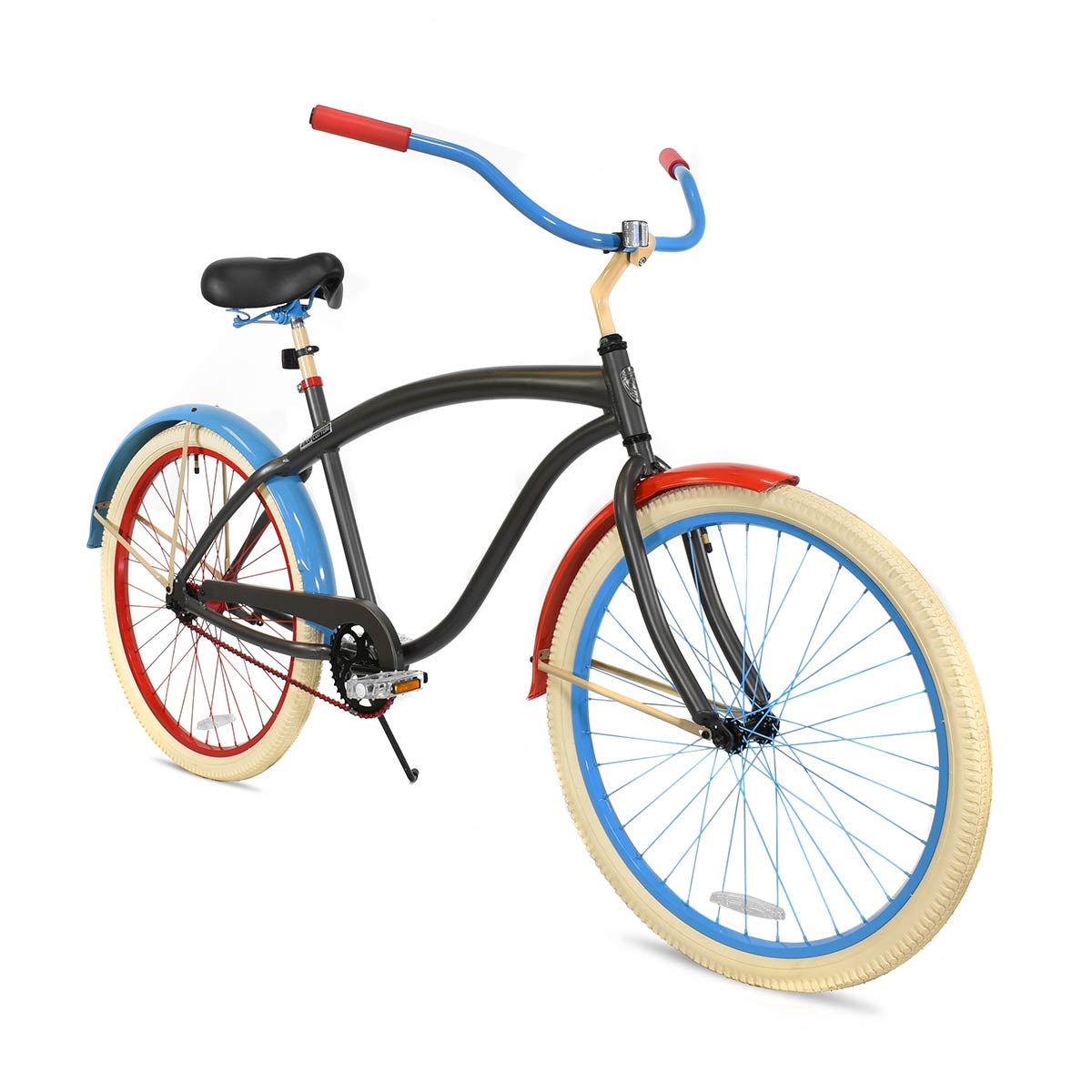The image depicts a child's bicycle designed for a 5- to 6-year-old, featuring a striking combination of black, red, blue, and creamy beige hues. The main frame of the bike is predominantly black, accompanied by a black seat and chain, highlighting its vibrant accents. The front wheel showcases a blue rim with matching blue spokes, while the back wheel contrasts with a red rim and red spokes. Both tires are cream-colored. The handlebars are primarily blue, adorned with red grips at the ends. Additionally, a red frame encloses the front tire, and a blue frame adorns the rear tire. The bicycle also includes a small kickstand and a pedal reflector, resting against a plain white background and aimed toward the bottom right angle in the photograph.